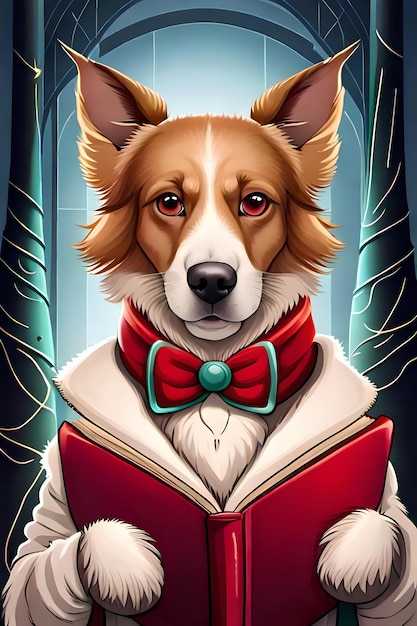The image depicts an animated, highly detailed AI drawing of a border collie dog, attentively reading an open red book. The dog has a brown head with long, pointy ears, red eyes, and a black nose, and his white muzzle contrasts sharply with his expressive face. A thick red bow tie, trimmed in green and resembling a nascot, wraps around his neck, adorned with a small gold chain that dangles slightly. He is dressed in a high-fur-collared jacket with large, crinkled lapels resting on his front legs, which are raised to hold the book open, one paw on each side of the white pages. The background features an arch framed by two teal trunks that bleed into emerald green with silver lines, giving the scene an elegant, almost regal atmosphere. The overall coloration includes shades of white, light green, and dark green, creating a bright and clear setting that enhances the detailed portrayal of the dog and his scholarly demeanor.